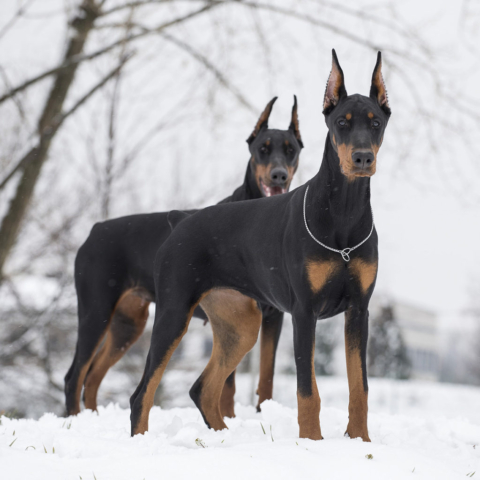This photograph depicts two majestic Doberman Pinscher dogs standing in a snowy field on a winter day. Both dogs, with their black and brown coats, are centered in the image, positioned one behind the other in a staggered manner. The dog in the foreground is closest to the viewer, showcasing a sleek side profile with its head turned to the right, adorned with a silver-gray collar. Behind it, the second Doberman also displays a side profile with its ears pointed upwards and its mouth slightly open, revealing red and white teeth. The ground is blanketed in white snow, while the top left background features bare brown trees with branches devoid of leaves, typical of the winter season. The overall scene captures the elegance and poise of the Dobermans against a serene, wintry landscape.